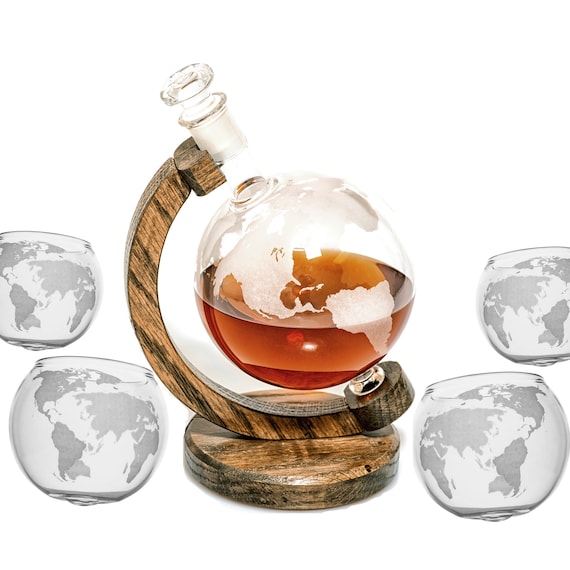The image showcases an elegant drinkware set against a plain white background, featuring a glass globe decanter filled with an amber-colored liquid, likely whiskey. The decanter, designed to resemble a globe with frosted white etchings of the world's continents, is supported by a light brown wooden stand with a circular base. The stand has an arc-shaped piece curving from right to left, holding the globe aloft. Surrounding the central decanter are four matching clear glasses, each etched with the same globe design, displaying different views of the Earth: North America and South America on one, and Africa, India, and Eurasia on the others. The detailed craftsmanship of the set exudes a sophisticated charm, making it an ideal gift for enthusiasts of fine spirits and geography alike.